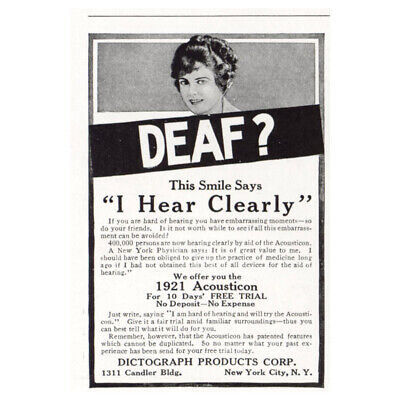This is an old black-and-white newspaper or magazine advertisement clipping on off-white ivory paper. The advertisement prominently features a photograph of a woman with short, dark curly hair pinned up around her head, displaying only her face and neck. Directly underneath the photograph, a black bar features white text in all caps reading "DEAF?" Below this bar, in black text, it states, "This smile says, 'I hear clearly.'" Smaller, less legible paragraphs follow these statements. The advertisement also includes a line in larger text that reads, "We offer you the 1921 Acousticon for 10 days free trial, no deposit, no expense." At the bottom, there is an address for Dictograph Products Corp, located in New York City, New York.